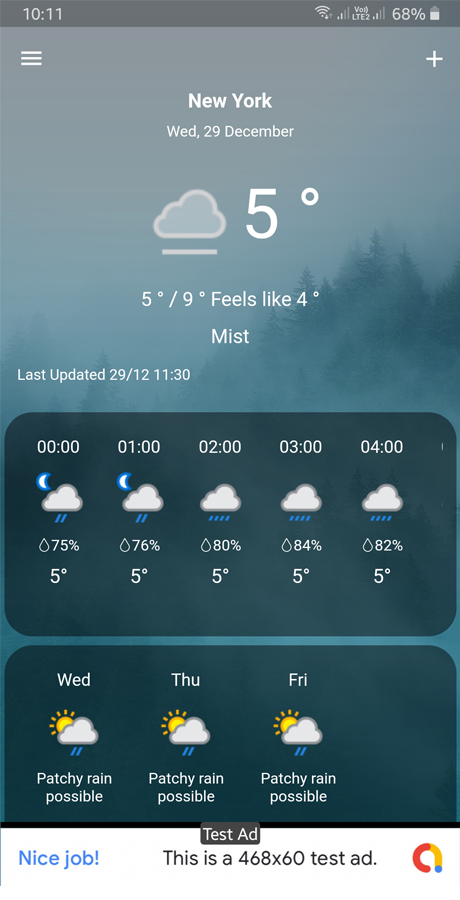Screenshot of a weather app showing the current forecast for **New York** on **Wednesday, 29th December**. The backdrop features a stormy mountain scene. At the top, it displays the location name and date, followed by a cloudy icon denoting a temperature of **5°C**. 

Directly below, it notes a range of **5°C / 9°C**, with a "feels like" temperature of **4°C**, and a condition described as "mist." Information indicates it was last updated on **29/12 at 11:30**.

Hourly forecasts run from 00:00 to 04:00, each accompanied by cloudy icons with rain. The respective chances of rain are **75%**, **76%**, **80%**, **84%**, and **82%**, consistently showing a temperature of **5°C**. Further details indicate the next rain probability drops to **10%**.

Another section highlights daily forecasts for **Wednesday**, **Thursday**, and **Friday**, each presenting a rain cloud with the sun peeking out, labeled as "Patchy rain possible."

In the top-left corner, the time reads **10:11**.

At the bottom, a white bar features a test advertisement, with the text: "Nice job! This is a 468x60 test ad," accompanied by a multicolored logo with red, yellow, and a blue dot on the right side.